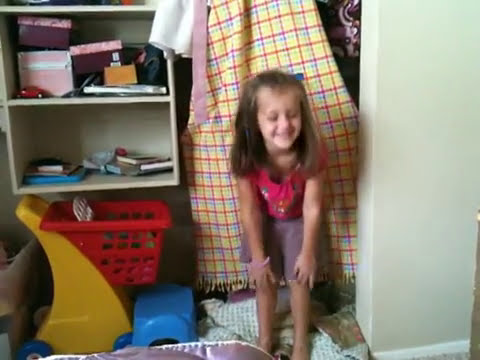The photo captures a delightful moment in the bedroom of a young, white girl around five years old. She has long brown hair styled into two pigtails and is dressed in a red shirt and brown skirt. The girl is standing up, bending over with her hands near her knees, laughing or smiling. The room is somewhat cluttered, reflecting a typical child's space with various items scattered around. 

To the left of the girl, there is a white bookcase with two shelves. The shelves are filled with books, DVDs, boxes, and a small toy car. Underneath the bookcase sits a red plastic basket on top of a yellow and blue children's shopping cart toy. The background includes a red and yellow plaid towel hanging up and a beige or gray wall to the right. The flooring has soft coverings, adding to the cozy atmosphere of the room. The girl appears energetic and joyful, epitomizing the playful innocence of childhood.